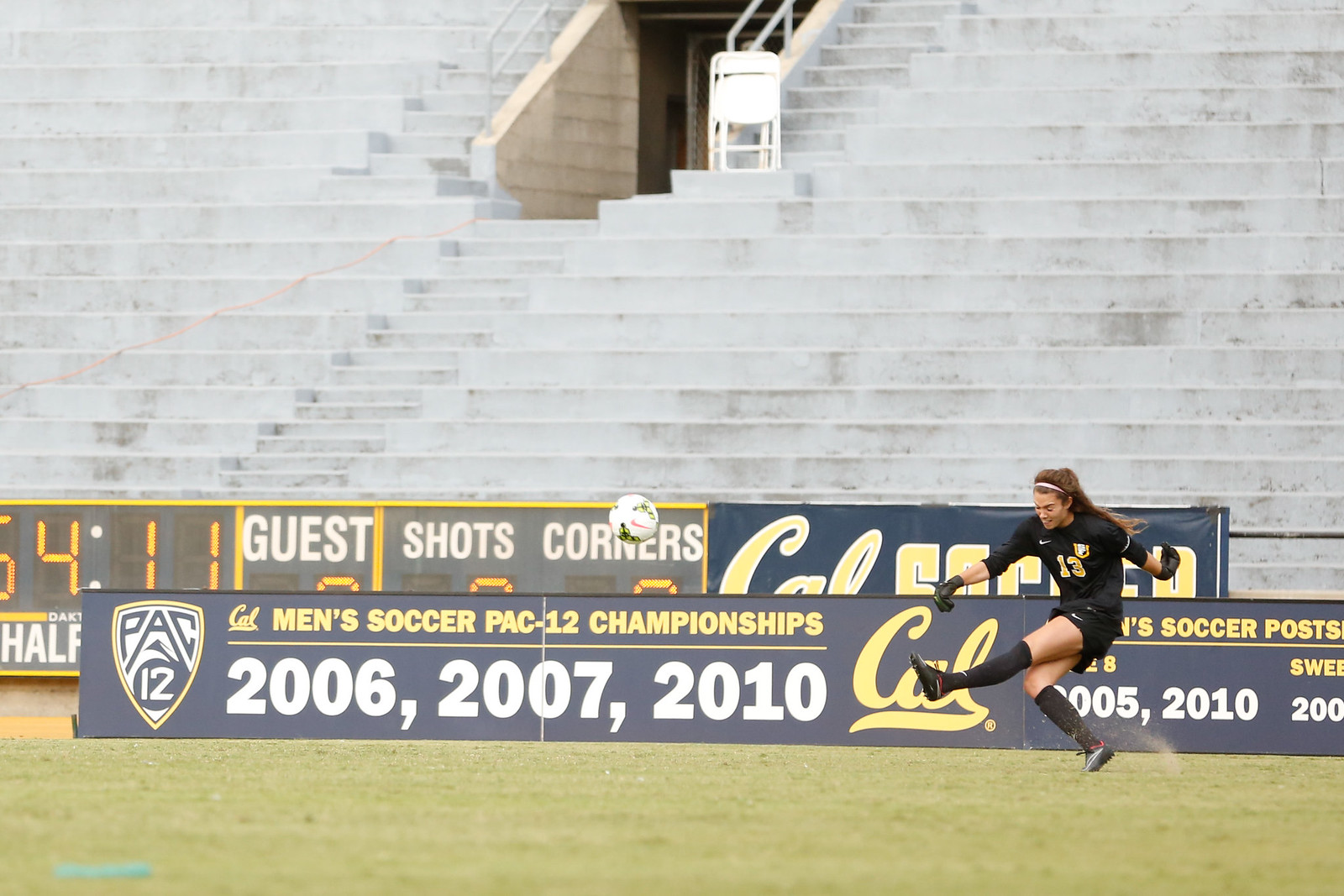In this full-color daytime photo, a young woman dressed in a black soccer outfit including black gloves, black knee-high socks, and black cleats, is captured mid-air after kicking a soccer ball, which is no longer in the frame, indicating a powerful kick. She sports a light headband over her light brown hair and a yellow number on her jersey. The scene is set on a bright green soccer field, likely at Cal State, as suggested by the prominent Pac-12 sign displaying the “Men's Soccer Pac-12 Championships” from the years 2006, 2007, and 2010. Behind her, you can see the lower walls leading up to gray concrete seats and steps, part of a larger stadium structure with a central entryway. A digital scoreboard shows “54” and “11,” alongside sections labeled "Guest," "Shots," and "Corner," though these details are partially obscured by the championship sign.